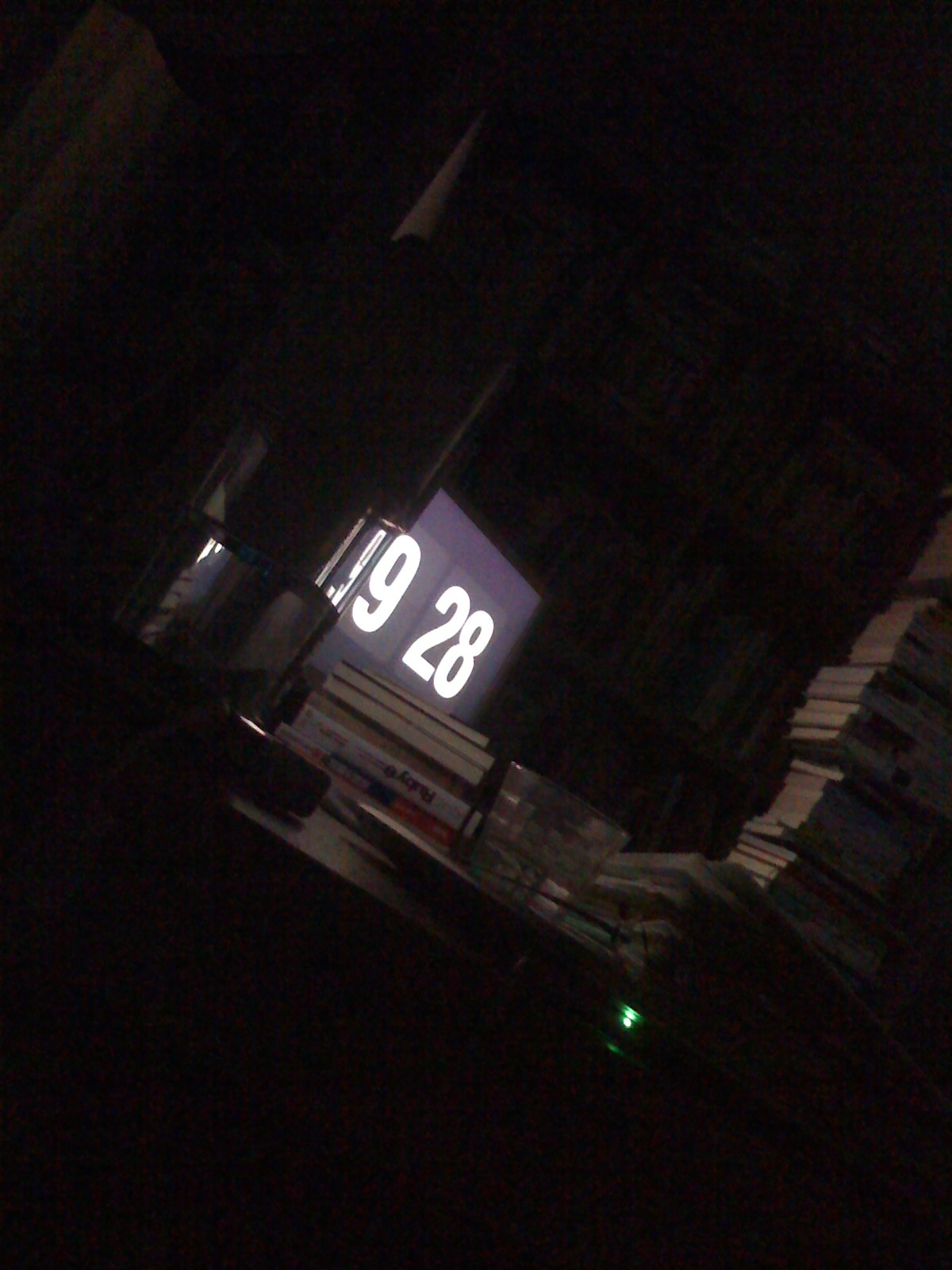In a dimly lit room, likely somebody's bedroom or perhaps even a library, a desk is illuminated by a bright digital clock. The clock, displayed on a slanted monitor or TV screen, shows the time "9:28" in large white numbers against a black background. To the right of the screen, there are tall stacks of books, with another smaller stack close by. A glass, potentially on a plate, sits among the items, emitting a small green light from an unidentified source nearby. The overall image is very dark, with faint outlines of a bookshelf and other indistinguishable items visible in the background, adding to the room's low-light ambiance.